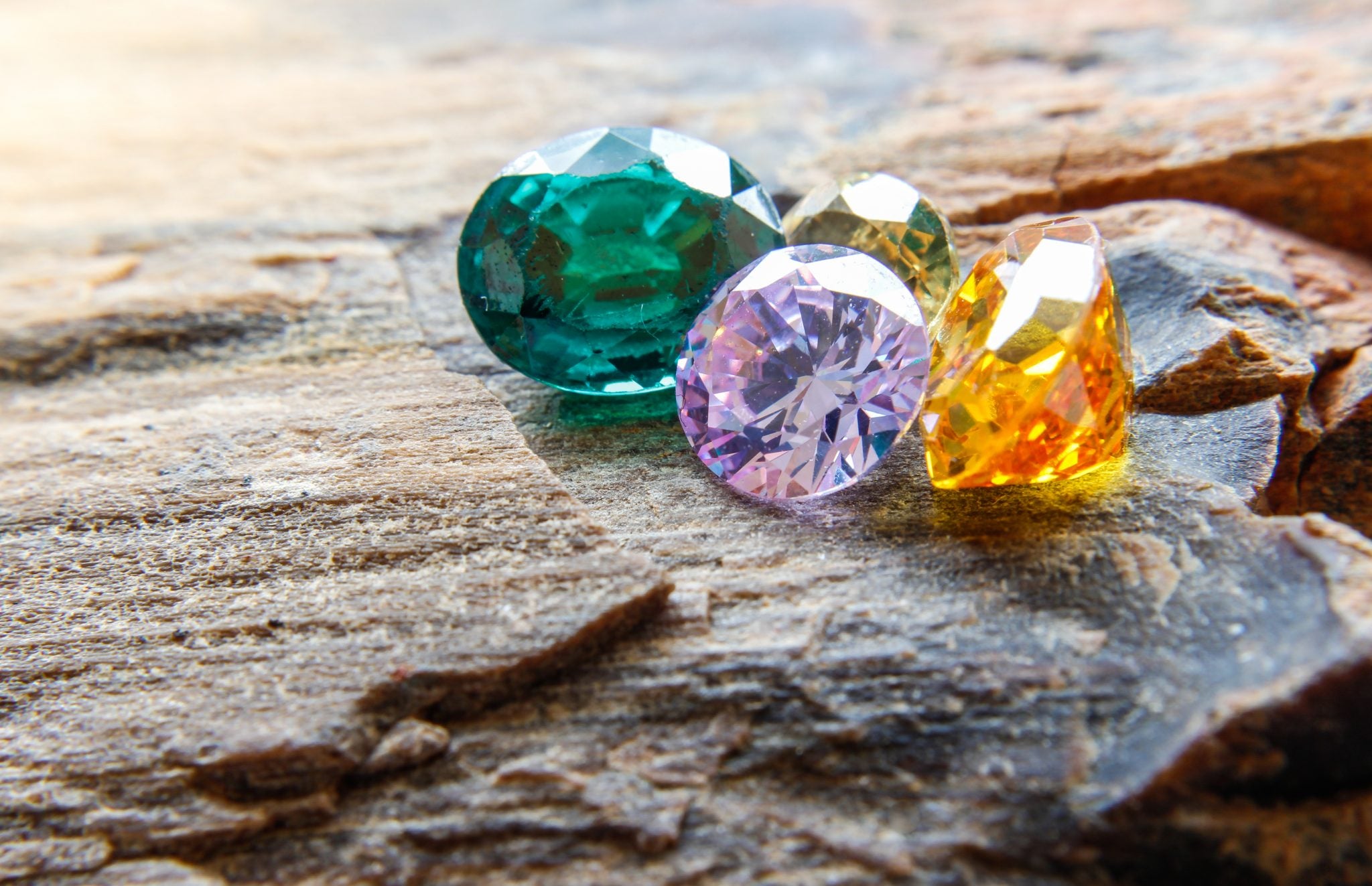This captivating outdoor photograph, taken in natural daylight, features a cluster of four brilliantly colored gems arranged on a rugged slate substrate by a water shore. Prominently positioned at the center of the image, the gems include a striking pink diamond, an emerald-green gem, an orangey-yellow diamond, and a light-colored diamond. The rocky slate surface, characterized by shades of black, white, gray, and tan, extends to the water's edge, evoking a mountainous landscape. The image, devoid of any text, highlights the unique colors and brilliance of the gems, which sparkle in the natural sunlight, adding an enchanting allure to the serene outdoor setting.